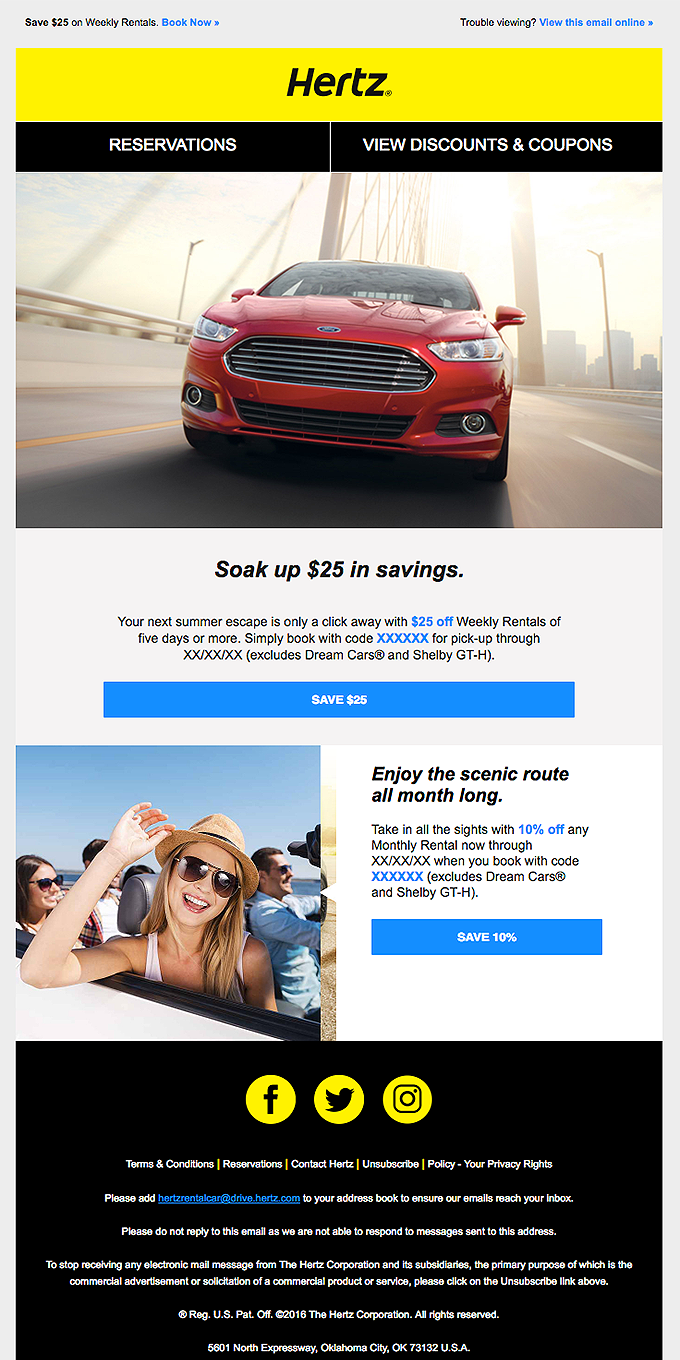This portrait-oriented advertisement by Hertz Car Hire features a well-structured layout, encouraging users to book their next rental. At the top, there's a small font section for browsing options such as "Book Now," "View Site," and "Email Online." Below, a prominent yellow bar stretching nearly edge-to-edge showcases the Hertz logo in black italics.

Underneath, two black tabs stand out, one labeled "RESERVATIONS" and the other "VIEW DISCOUNTS AND COUPONS," both in white uppercase letters. The centerpiece of the ad is an image of a sleek red Ford car cruising over an unidentified suspension bridge.

Following the image, the advertisement text reads: "Soak up $25 in savings. Your next summer escape is only a click away with $25 off weekly rentals of five days or more. Simply back with code [placeholder] for pickup through [placeholder]." Accompanying this text is a blue button that states "Save $25."

Near the bottom, there's a picture of a cheerful lady wearing dark glasses, a straw hat, and a sleeveless white top. She has long blonde hair and is enjoying the ride with four other passengers. Next to this engaging image, a text section reads: "Enjoy the scenic route all month long. Save 10%." 

This comprehensive setup entices potential customers with significant savings and the joy of scenic travel experiences.